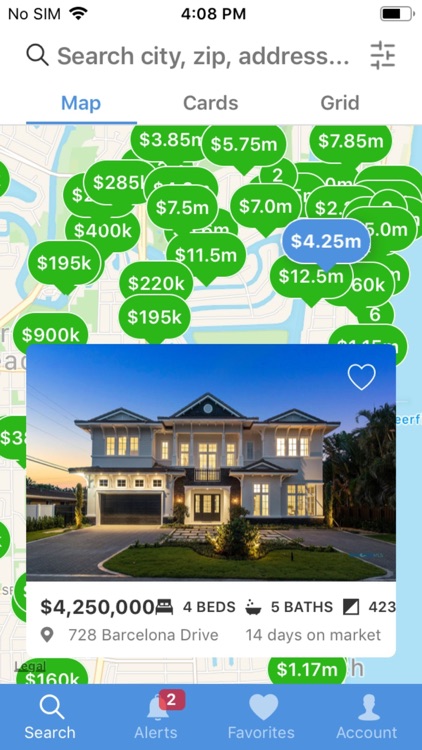This is a detailed screenshot of house hunting results. Centrally, there is a large map dotted with pins representing various properties. These pins, resembling text bubbles with rounded edges, are primarily green with white prices prominently displayed, ranging from $195k to multi-million-dollar listings. One pin on the right stands out with a blue background, indicating a selected property.

Below this selected pin, there is an image of a well-lit, attractive house against a backdrop of a dark blue sky, suggesting a sunset on the left side. The house features a manicured lawn, a spacious garage, and a well-maintained pathway. 

Adjacent to the house image, the price is listed as $4,250,000. Additional information specifies the property has four bedrooms and five bathrooms, though part of the text reading "423" is cut off, obscuring its context. The address is clearly visible as 728 Barcelona Drive, and it's noted that this house has been on the market for 14 days.